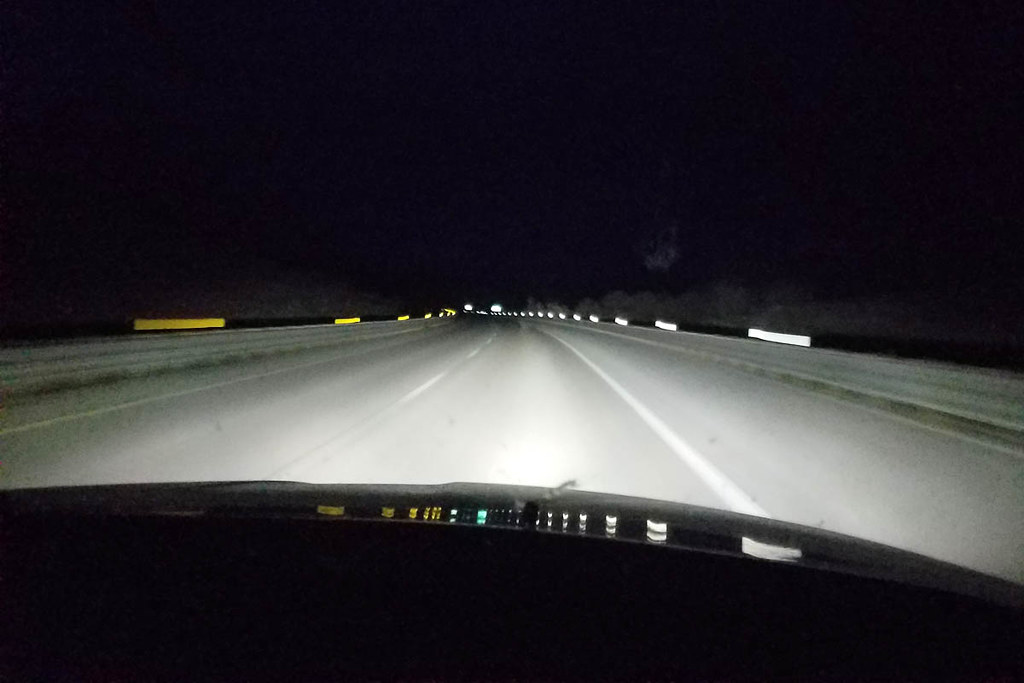A nighttime photograph taken through the windshield of a moving car. The dark dashboard frames the bottom of the image, with faint reflections where the windshield meets the back dashboard, partially outlining the car's front interior. The sky appears grainy and pitch black, suggesting the use of a flash that washes out some details. On the right side, a metal guardrail with a black stripe and white lights is visible, illuminated against the dark backdrop. The highway median, marked by a curving white line, guides the view forward, with white center lines clearly dividing the lanes. To the left, another median features a black metal guardrail adorned with yellow reflectors, and faint, blurry outlines of trees line the road. The overall scene is slightly blurred, capturing the sense of movement.